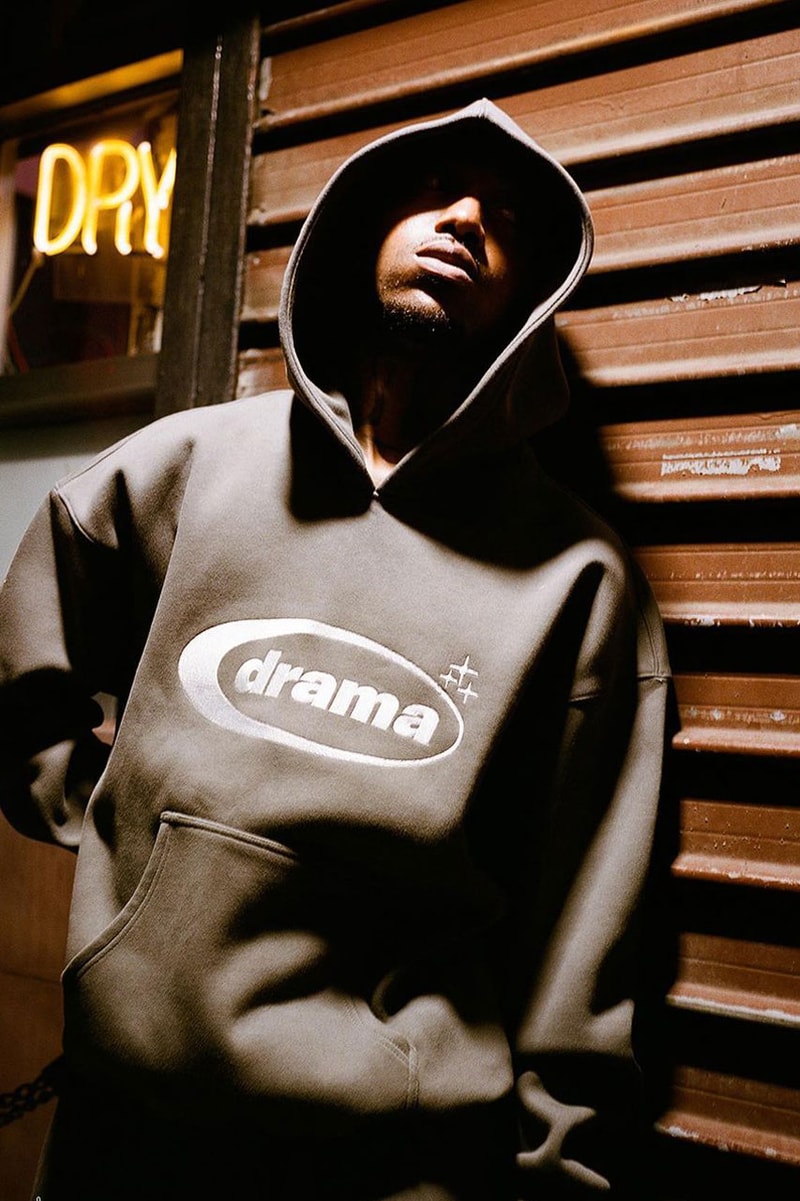This photograph features an African-American male wearing a gray or black hoodie adorned with a circular logo containing the word "drama" in lowercase white letters. The logo's circle is designed with varying thickness, getting wider as it moves from right to left, and is accompanied by three small star-like crosses on the right side. The hoodie also has a kangaroo pouch in the front. The man is leaning against a brown, sectioned pull-down door that resembles a garage door. He has short facial hair on his chin and his hood is pulled over his head, obscuring his eyes as he looks slightly upwards to the left. His hands are relaxed by his sides. Above the man, to the top left, there is a neon yellow sign that reads "DRY".